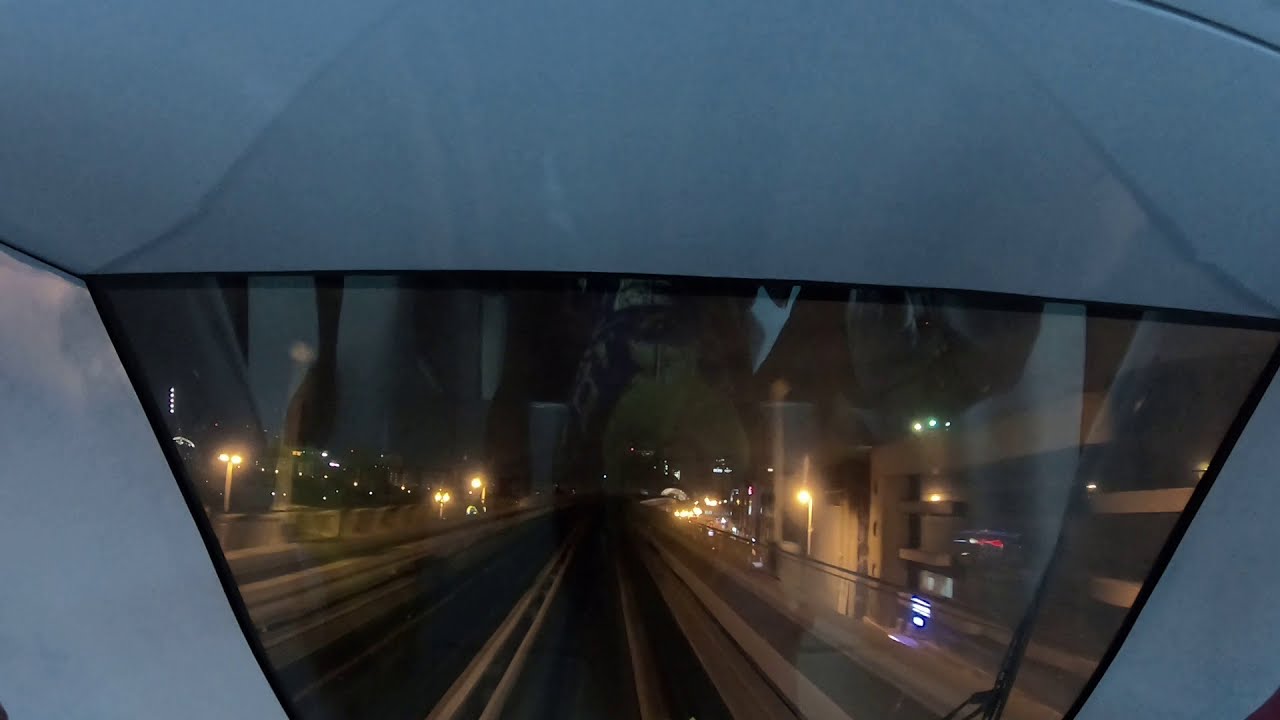This full-color nighttime image, rectangular in shape without any borders, seems to have been captured from the front window of a high-speed rail train or tram, possibly of Asian origin such as a Shinkansen or a Chinese bullet train. The window, bordered by light-colored plastic, offers a clear view of the illuminated rail tracks extending outward, framed by railings and lit lamps. On the right side, buildings are visible, one of which displays red signage, suggesting an area that could be an airport or a bustling urban landscape. Reflections of people inside the train are faintly visible on the window, enhancing the sense of motion. Additionally, a window wiper is parked on the right, further suggesting the viewpoint is from the front of the train. The overall scene intimates a high-speed journey through a vibrant, lit-up cityscape at night.